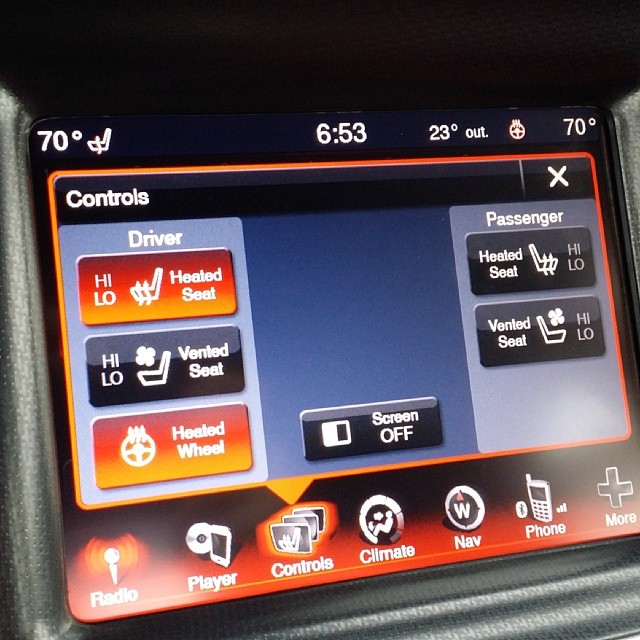This image captures a digital control screen inside a car, featuring a variety of controls and icons for the vehicle's interior settings. The background of the screen is predominantly black, with text and icons in white, red, and orange. In the top left corner, it shows the interior car temperature at 70 degrees, accompanied by a seat belt indicator. The top middle part displays the time as 6:53, with the exterior temperature listed as 23 degrees, and again 70 degrees for the interior temperature on the top right.

The central portion of the screen is bordered in orange and contains several control options. On the left, labeled "Driver," there are buttons for high and low heated seats, high and low vented seats, and a heated steering wheel. On the right, labeled "Passenger," similar options are available for heated and vented seats. A prominent "Screen Off" button is located in the middle of these controls.

At the bottom of the screen, various icons represent different functions: a microphone for radio, a CD for the player, a person sitting for climate control, a compass for navigation, a phone icon, and a plus symbol for more options. The overall interface is designed to provide a comprehensive control hub for the car's interior environment.